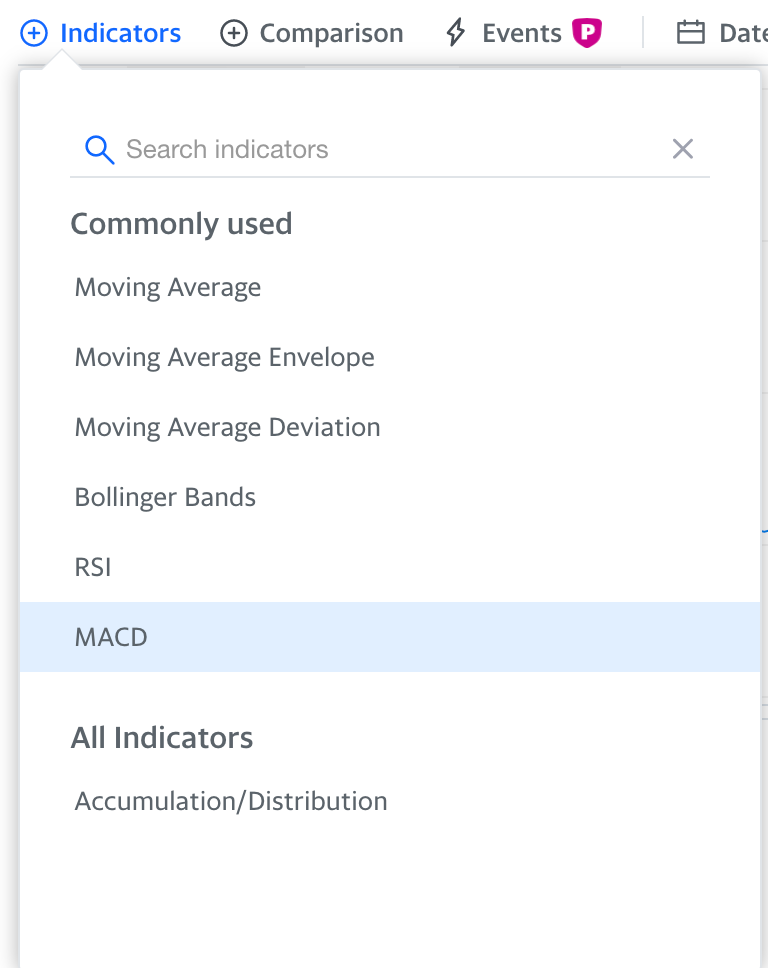This is a detailed screenshot of an informational menu interface. At the top of the menu, there are several categories listed: "Indicators" in blue text, followed by "Comparison" in black text. To the right of "Comparison," there is another black-text label, "Events," which is accompanied by a lightning bolt icon. Additionally, there is a distinctive purple icon with a white letter "P" in the center, next to a category labeled "Data."

Below these primary categories, the menu includes a search bar labeled "Search Indicators," which features a magnifying glass icon and an "X" for closing the search option. The subsequent section is labeled "Commonly Used" and includes a list of popular analytical tools: "Moving Average," "Moving Average Envelope," "Moving Average Deviation," "Bollinger Bands," "RSI," and "MACD."

Further down, the menu has a section labeled "All Indicators," and the text "Accumulation/Distribution" is visible, likely indicating options for deeper analysis or additional tools within the menu.